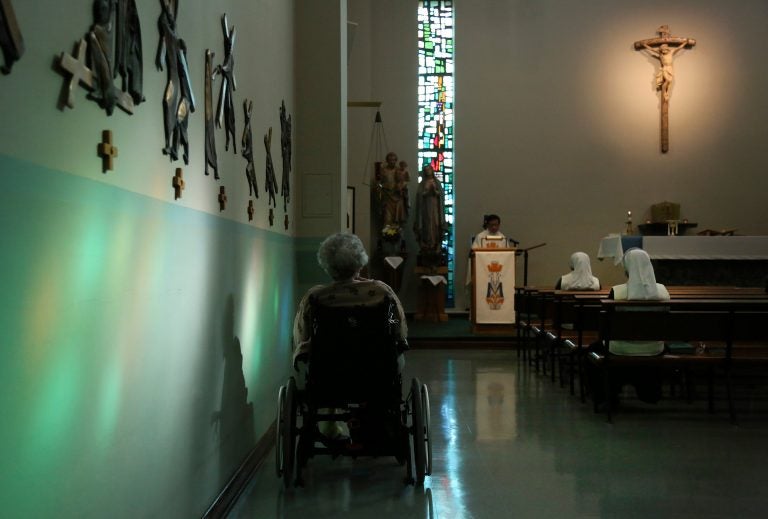This full-color photograph, taken indoors with both natural and artificial light, captures an intimate moment inside a church. The image, square in composition, has a visually striking polished floor reflecting the serene atmosphere. The left side of the scene features a white and blue wall adorned with several crucifixes and religious figures, leading the eye towards the center, where a large stained glass window and carved saints stand prominently. In the foreground center-left, an older lady with gray hair sits in a wheelchair, absorbed in the sermon. To the center right, two nuns dressed in white occupy the wooden pews, attentively listening. At the front, a speaker stands behind a white lectern, delivering the sermon. The top right features a crucifix with Jesus, illuminated by a warm, yellow halo of light, emphasizing the sanctity of the setting. The hues of blue, green, pale red, beige, tan, and white blend harmoniously to encapsulate the decor of this solemn church interior.